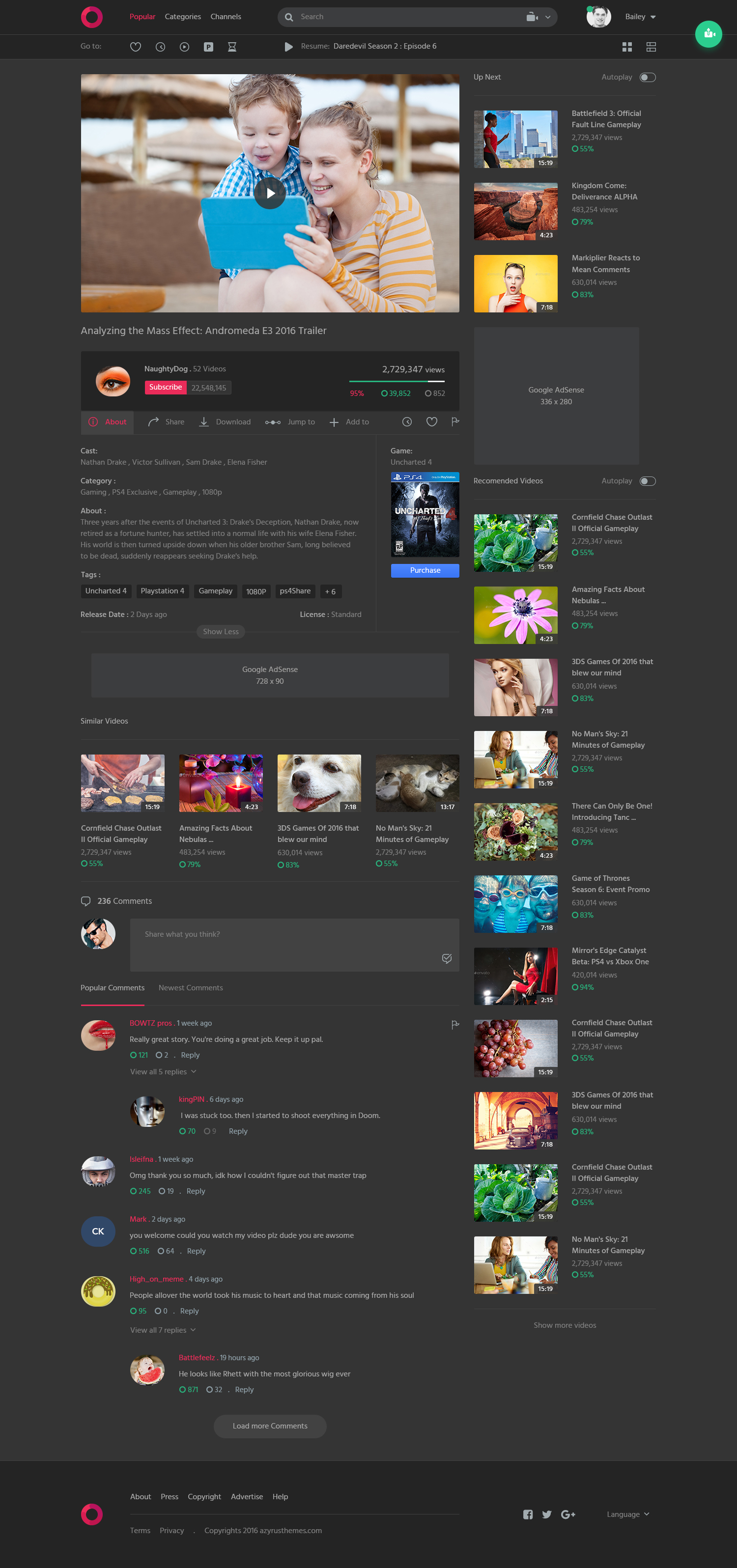The image is a detailed screenshot with a dark grey background, featuring a user interface. At the top left corner, a hot pink circular logo is displayed. Adjacent to the logo are menu options: "Popular" written in hot pink text, followed by "Categories" and "Channels" in white text. To the right of these options is a search bar with no input, and next to the search bar are icons of a video camera and a profile picture of a fair-skinned male identified as Bailey.

Below this, a toolbar offers several options: "Go To," a heart icon, a clock icon, a circular icon with a play button, a square icon with the letter "P," an hourglass icon, and a play button labeled "Resume, Daredevil Season 2 Episode 6."

Beneath the toolbar is a large video screen grab showing a fair-skinned woman and child sitting together, focused on a tablet. To the right of the screen, there is a "Up Next" list featuring video titles: "Battlefield 3 Official Faultline Gameplay," "Kingdom Come Deliverance Alpha," "Markiplier Reacts to Mean Comments," a collection titled "Naughty Dog 52 Videos," and another titled "Analyzing the Mass Effect, Andromeda E3 2016 Trailer."